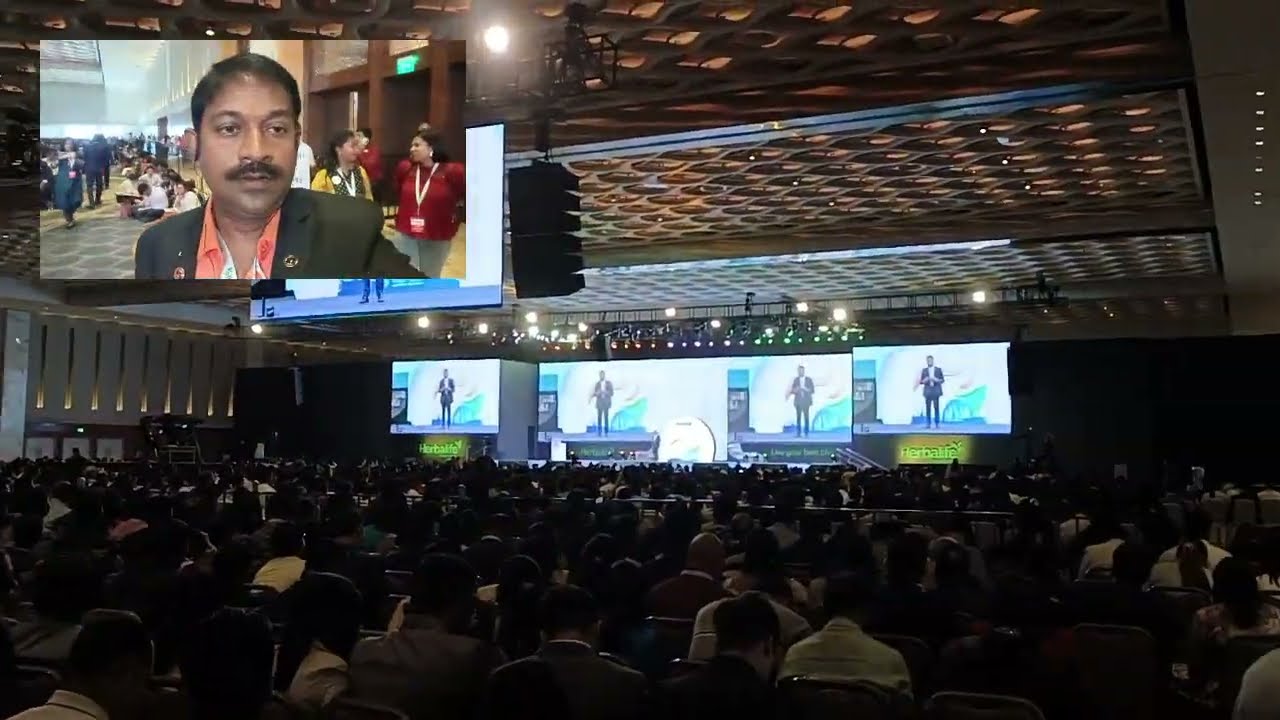The image depicts a large auditorium filled with attendees, all facing multiple large screens at the front of the room, each displaying images of a man. The stage is illuminated with lights, and several screens show a man who appears to be the focal point of the presentation. This man, difficult to distinguish clearly on the distant screens, is portrayed in an inset image in the top left corner. Here, he is seen walking through a hallway crowded with people wearing lanyards, suggesting a conference or similar event. He is an Indian man dressed in a black jacket over an orange shirt with an open collar, sporting short black hair and a bushy mustache. The auditorium itself is darkened, with overhead lighting and additional screens suspended from the roof, ensuring visibility for those seated farther back. The words "Herbal Life" are visible on the screens, indicating that the event is likely related to this organization.